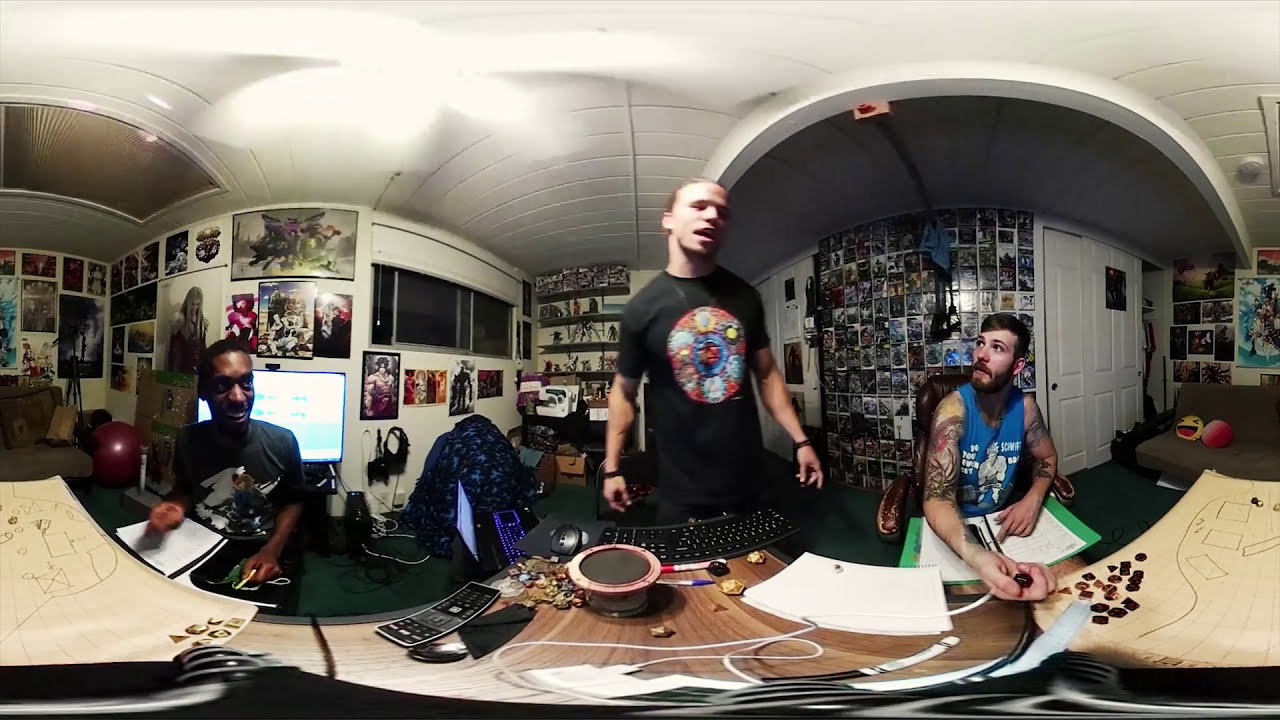This panoramic photograph captures a busy, detailed scene of three men in what looks like a recording studio. The focal point features three men: a black man on the left wearing a black t-shirt, a standing man in the center also in a black t-shirt with a multicolored symbol, and a white man on the right in a sleeveless turquoise shirt with tattoos on his arms. The men are positioned around long, brown tables cluttered with various items including sheets of paper with pencil sketches of top-down building views, drawing utensils, a keyboard, pens, pencils, a phone, and other tools. The man in the center appears to be talking, possibly into a microphone descending from the ceiling, while the man on the right seems to be counting change or tokens on a piece of paper. The background reveals a rounded room with a scalloped roof, showcasing walls adorned with numerous photographs, posters, and other artwork. There are shelves with possible collectible action figures, a medicine ball on the far left, a couch on the right, and white doors on either side of the arched area transitioning into another room, completing the scene's intricate details and vibrant atmosphere.